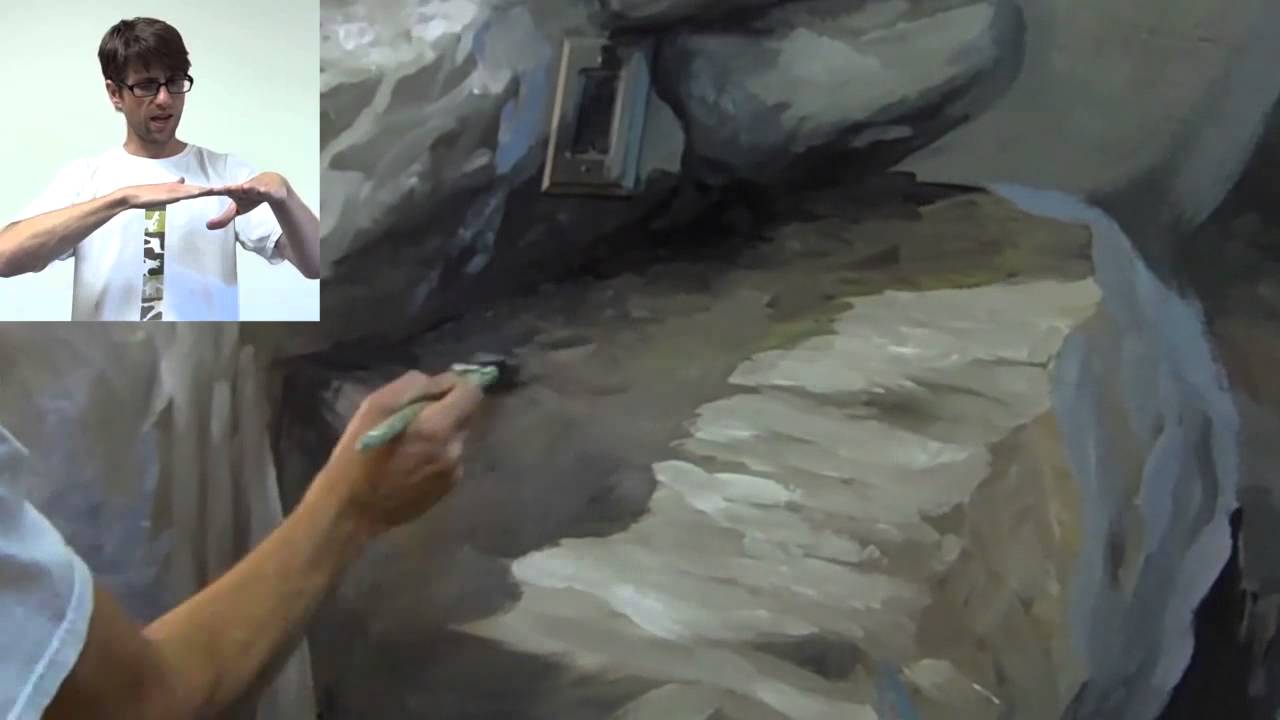This photograph captures an artist in the process of painting a detailed image of large gray boulders. The artist’s arm is prominently featured, leaning forward with a green brush as they add intricate details and shadows to the partially completed painting of rocks. The focus is entirely on the hand and brush, as the photo is cropped just below the shoulder. The overall color scheme of the painting includes various shades of gray, creating a realistic portrayal of the rocky textures.

In the top left corner of the image, there is a small screen overlapping the main photo, which appears to be a paused video. This screen displays a man with brown hair, wearing brown eyeglasses and a white t-shirt, gesturing with his hands, possibly explaining the painting process. The man’s clothing matches the attire of the person painting, suggesting they are the same individual captured at different moments – one in the act of painting and the other providing a detailed explanation of the technique. The image is devoid of any accompanying text.